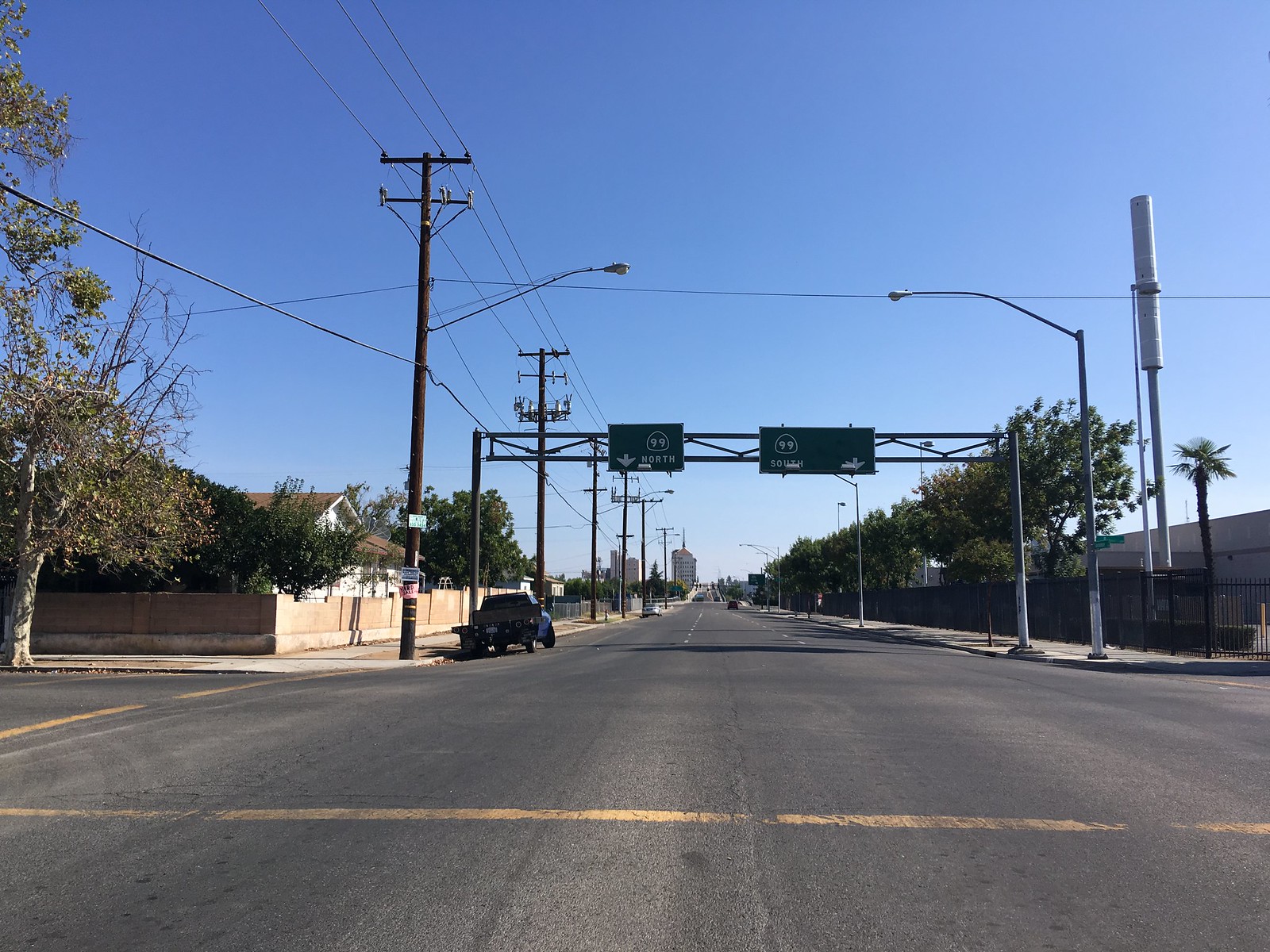This photograph captures a busy street intersection surrounded by various urban elements on a clear day. On the left-hand side, a half-bare tree, with exposed branches jutting out from its upper portions, stands prominently. Below this tree, a yellow cement wall with a white base lines the sidewalk, providing a boundary for more trees and a house behind it. Adjacent to the tree, a blue truck partially enters the frame, parked beside a street lamp adorned with an array of power lines that extend across the street.

Overhead, a large green street sign directs traffic with indications for 99 North and 99 South. This sign marks the intersection, which is framed by another light pole on the opposite side. This pole stands near a metallic fence and a building that appears set back from the road. Looking further down the street, you can observe additional buildings lining the horizon, creating a layered urban vista.

In the foreground, the bottom edge of the photograph reveals the paved street, clearly demarcated by yellow lines guiding vehicular flow. The composition, with its mix of natural and man-made elements, offers a snapshot of a typical yet intricate cityscape scene.